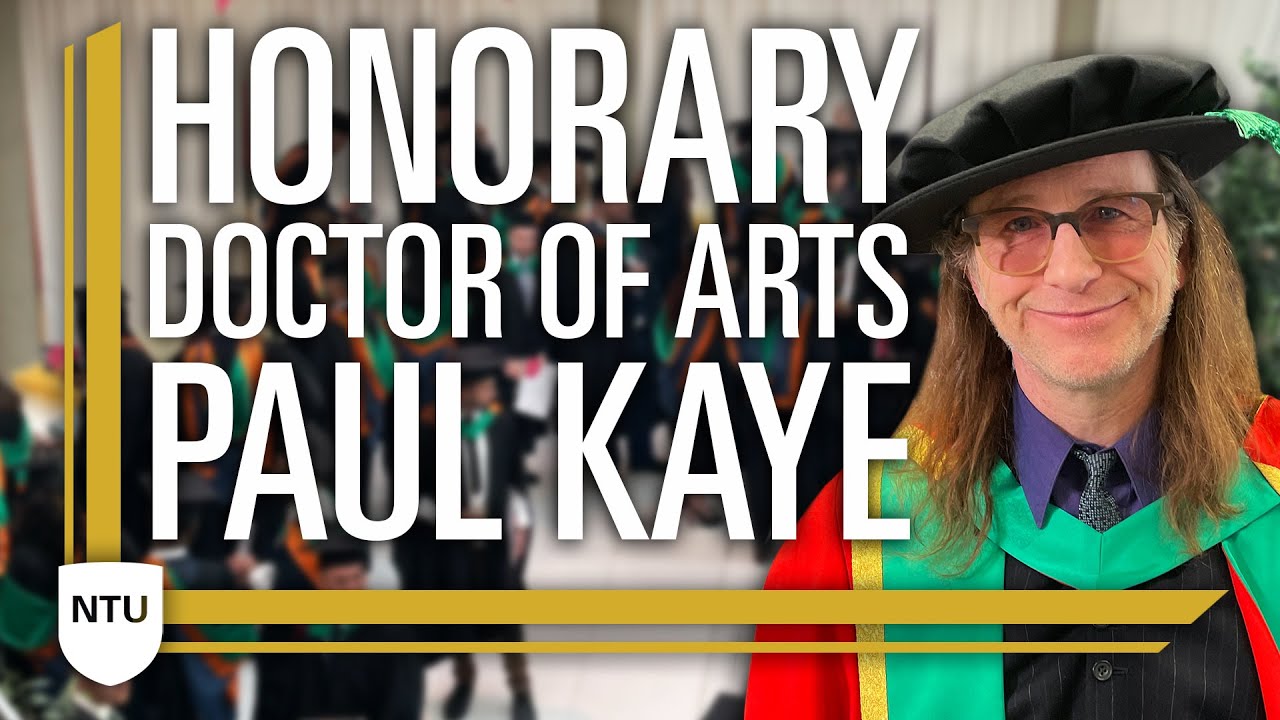The image depicts a celebratory poster or flyer, prominently featuring a joyous moment of recognition. Central to the composition, on the right side, stands a man identified as Paul Kaye, who has been awarded the title of "Honorary Doctor of Arts." Paul Kaye, exuding happiness, is adorned in a graduation gown that stands out with its intricate and vibrant detailing. The gown features red sleeves, a green scarf, and yellow stripes. He also wears a blue button-up shirt and a matching blue tie. His head is crowned with a large, round black hat adorned with a green ribbon on the left side. His long, flowing brown hair reaches his shoulders, and he sports reddish-tinted glasses, framing his beaming face.

In the background, the image captures a student body sporting similar graduation attire, indicating a celebratory academic setting, possibly a graduation ceremony, filled with joy and accomplishment.

Dominating the left side of the image are large white letters announcing "Honorary Doctor of Arts, Paul Hayes" from top to bottom. Complementing these elements, a bold yellow and deep green striped design adds a vibrant touch running vertically. In the bottom left corner, a white badge-like crest is prominently displayed, bearing the letters "NTU," and further emphasizing the academic achievement the image commemorates.